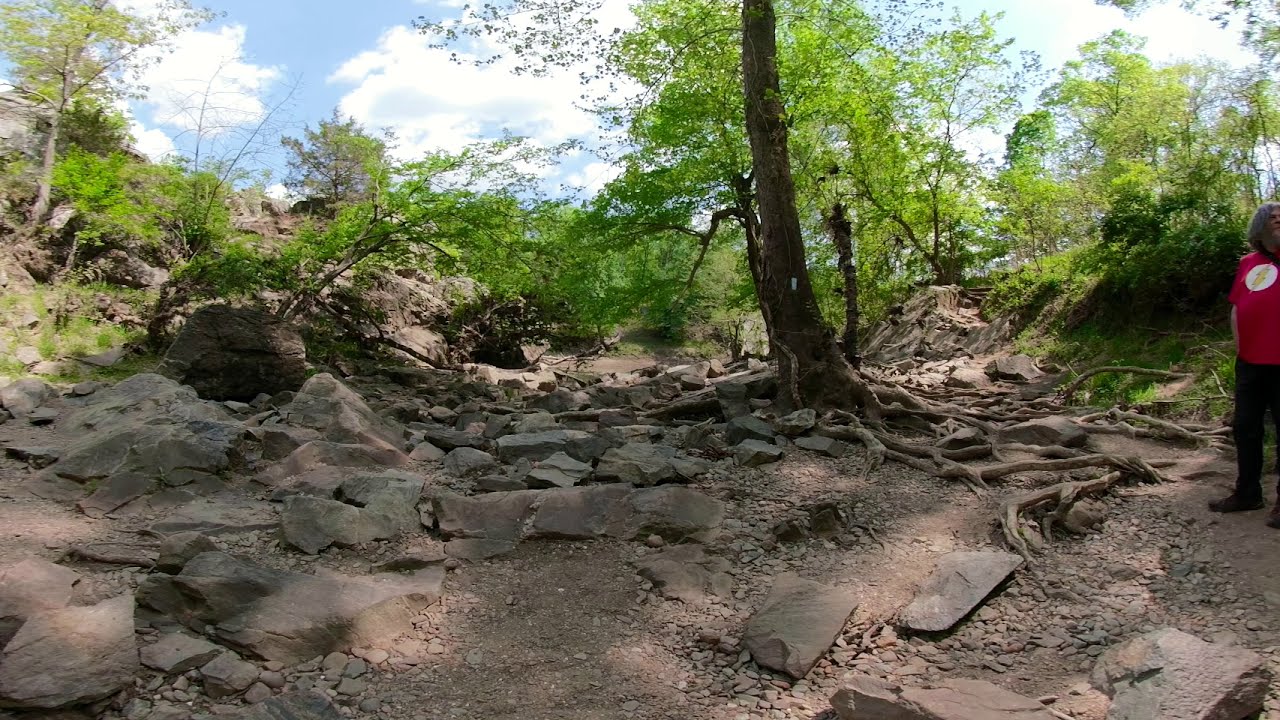The image captures a serene, sunny forest scene, likely during the spring or summer, evident by the vibrant green leaves on the trees. The foreground features a dried-up lakebed or riverbed, strewn with sand-colored rocks, pebbles, and larger flat stones. The landscape appears slightly bowed, suggesting a past flow of water. Centered in the image stands a large tree, while the background is filled with an array of other trees and lush shrubbery, creating a dense, healthy forest backdrop.

To the right side of the frame, a person is partially visible, standing and looking away from the camera. The individual, who appears to be in their 50s or 60s, is dressed in black pants and a distinctive red shirt adorned with the Flash logo—a white circle with a lightning bolt on the chest. The man also has long hair cascading down his back. Above, the bright blue sky is dotted with puffy clouds, and the sunlight filters through, casting dappled shadows across the rocky ground.